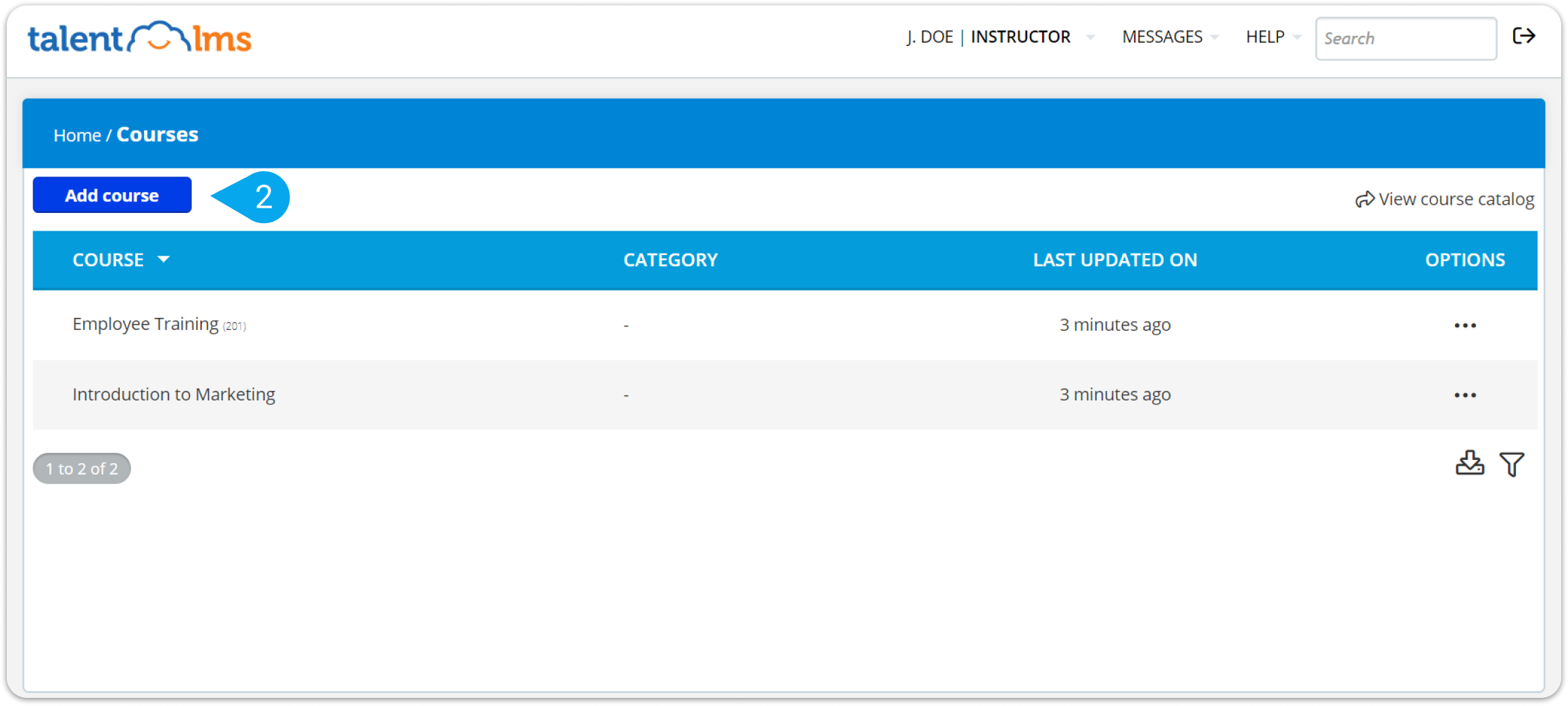This is a clear and detailed caption based on the description provided:

---

**Screenshot of Talent LMS Interface:**

This colored landscape-format screenshot showcases the Talent LMS software interface on a computer screen. The Talent LMS logo is prominently displayed at the top, featuring the word 'Talent' in blue and 'LMS' in orange, separated by a cloud-like shape. The profile belongs to J. Doe, an instructor, as indicated by the text near the logo.

In the top right corner, sections for 'Messages' and 'Help' are visible. Below, the interface shows a navigation path (Home/Courses) and an option to add new courses. Currently, two courses are listed: "Employee Training," last updated three minutes ago, and "Introduction to Marketing," also updated three minutes ago.

The page design is functional and straightforward, primarily using text with no images. A dark blue band highlights the 'Home/Courses' navigation, while a lighter blue band marks the course section headers, ensuring clarity and easy navigation.

---

This caption should provide a comprehensive description of the interface in the screenshot.